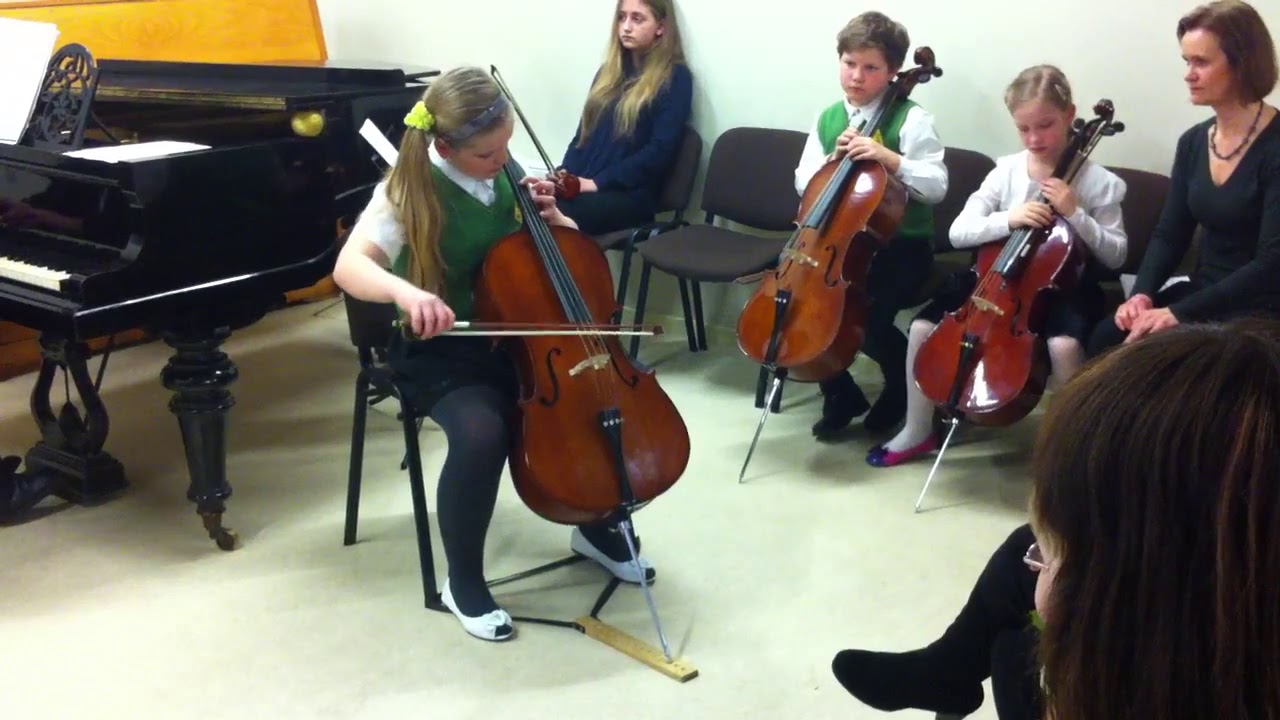In a brightly lit room of what appears to be a music school, a photograph captures a poignant moment of a young girl, roughly 10 years old, deeply immersed in playing a cello. Seated on a folding chair in front of a black grand piano, she is dressed in a green V-neck sweater vest over a white short-sleeved shirt, black tights, and white shoes. Her brown hair, tied with a ribbon into a side ponytail, cascades past her shoulders. 

To her right, along the yellow wall, sit three children and an adult. Closest to her is a blonde girl in black, sitting idly without an instrument, seemingly bored. Next is an empty seat, followed by a young boy, approximately 7 or 8, dressed in a green vest and black pants, holding a cello. Alongside him, a very young girl, around 6 years old, in a white sweater and black skirt with white tights, also holds a small cello. 

In the lower right corner of the image, a woman's face and legs are partially visible, wearing black tights. Her presence adds a subtle layer of adult supervision, possibly teachers or judges observing the performance. The golden floor softly reflects the scene, underscoring the ambience of disciplined yet heartfelt musical practice.